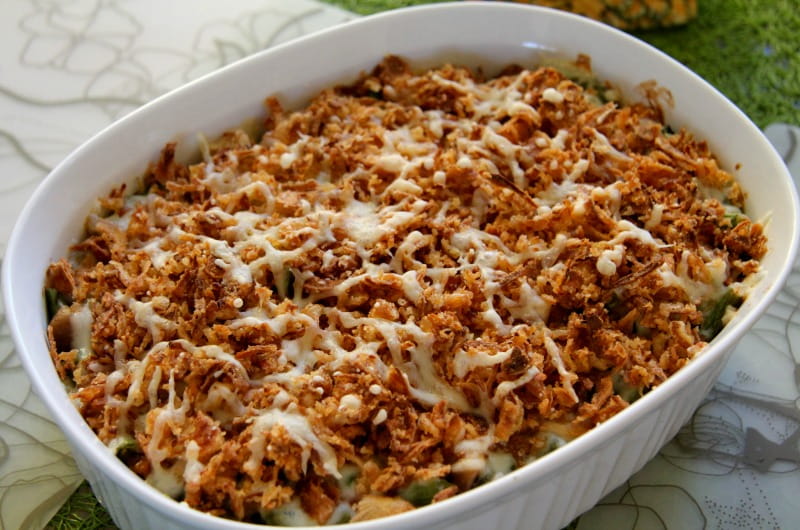The photograph captures a scene focused on a ceramic casserole dish that is white and slightly oval-shaped, featuring ridges on its sides for grip. This deep dish contains a layered, uneven mixture resembling pasta, sprinkled generously with both ground brown and white meats, and garnished with green vegetables that peek through from underneath. The food appears well-cooked with melted cheese melding seamlessly over the top. The dish sits on a table adorned with a white surface accented by gray lines and floral designs. The setting seems outdoors, evidenced by the patch of dark green grass visible in the upper right corner, illuminated by bright, natural light indicative of a sunny day. The overall composition of the photo is angled slightly from the bottom left to the top right, centering the attention entirely on the appetizing casserole. There are no people or text present in the image, enhancing the focus on the culinary display.